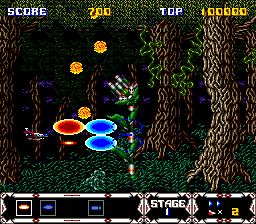This is a small, computer-generated image depicting a dense forest scene. On the right-hand side, a few tree trunks rise vertically, adding a touch of nature to the composition. The image is uniquely rendered with numerous tiny slots and strokes, rather than traditional pixels, providing an intricate, textured appearance. On the left side of the forest, three orange lights create a warm, glowing effect, while two large blue discs encircled by white also emit light, contributing to the enchanting ambiance. Additionally, one significant orange disc takes prominence in the scene. In the upper right-hand corner of the image, the word "Score" is displayed, followed by the number "700." Next to this, the word "Top" is visible alongside a counter, suggesting the image might be part of a game interface.